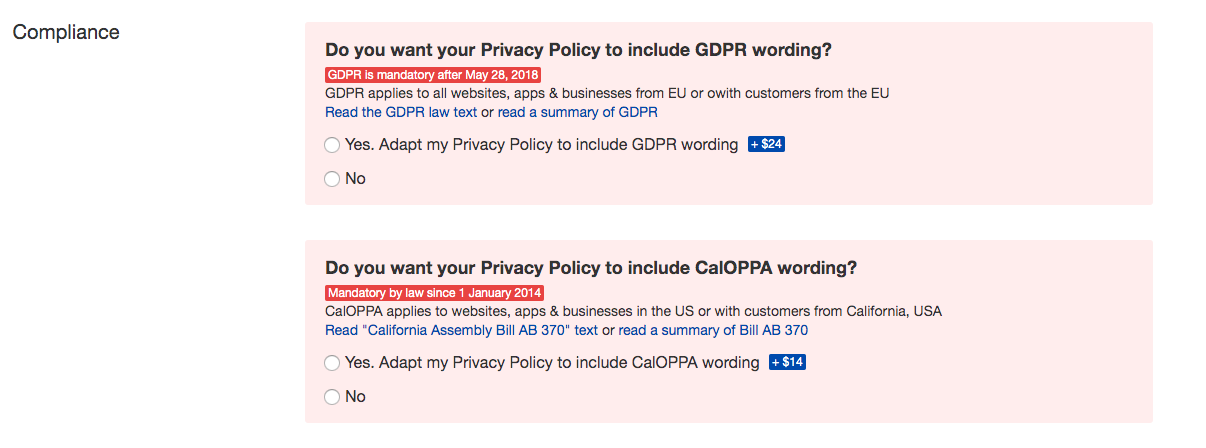The webpage presents options for updating a privacy policy in compliance with specific regulations. The page features a predominantly white background, with key sections highlighted in two rectangular boxes with pink backgrounds.

In the top-left corner, the page is labeled "Compliance." The first rectangular box addresses the inclusion of GDPR (General Data Protection Regulation) wording. It contains the following elements:

- **Black text on a pink background:** "Do you want your privacy policy to include GDPR wording?"
- **Reddish background text:** "GDPR is mandatory after May 28, 2018."
- **Pink background again:** "GDPR applies to all websites, apps, and businesses from the EU or with customers from the EU."
- **Link options:** "Read the GDPR law text" or "Read a summary of GDPR."
- **Selection circle for yes:** "Yes, adapt my privacy policy to include GDPR wording." The cost is displayed in a blue box, "Plus $24."
- **Selection circle for no:** An option that reads simply, "No."

Neither option has been selected in this section.

The second rectangular box focuses on the inclusion of CALAPA (California Privacy Protection Act) wording, and it contains the following elements:

- **Black text on a pink background:** "Do you want your privacy policy to include CALAPA wording?"
- **Orangish-brown background text:** "Mandatory by law since January 2014."
- **Pink background once more:** "CALAPA applies to websites, apps, and businesses in the US or with customers from California, USA."
- **Selection circle for yes:** "Yes, adapt my privacy policy to include CALAPA wording," with a price of "Plus $14."
- **Selection circle for no:** An option that reads simply, "No."

As with the first section, neither option has been selected here.

The detailed layout and color-coded sections effectively guide users through the choices for updating their privacy policies in line with GDPR and CALAPA regulations.